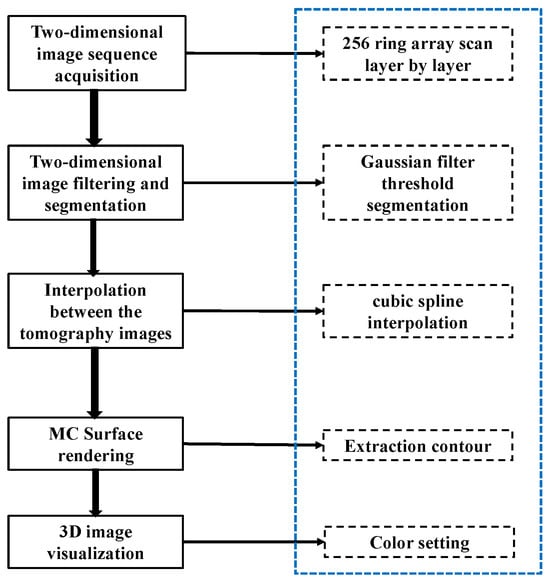The image displays a detailed flowchart with a series of interconnected rectangle boxes and arrows indicating the process flow. The chart is organized into two columns: the left column features five white rectangle boxes with black borders, sequentially arranged from top to bottom, while the right column features five boxes enclosed within a blue perforated box.

In the left column, the process begins with "Two-Dimensional Image Sequence Acquisition" at the top. A thick black arrow points downward to the next box, labeled "Two-Dimensional Image Filtering and Segmentation." Another arrow leads to the subsequent box that reads "Interpolation Between the Tomography Images." Continuing down, the next step is "MC Surface Rendering," followed by the final box in the column labeled "3D Image Visualization."

The right column, interconnected and running parallel, starts with "Two, Five, Six Ring Array Scan Layer by Layer." This is followed by "Gaussian Filter Threshold Segmentation," then "Cubic Spline Interpolation." The process continues with "Extraction and Contour," and concludes with "Color Setting."

The chart effectively illustrates a linear progression on the left side, accompanied by a detailed right column, both depicting a comprehensive workflow in image processing and visualization.